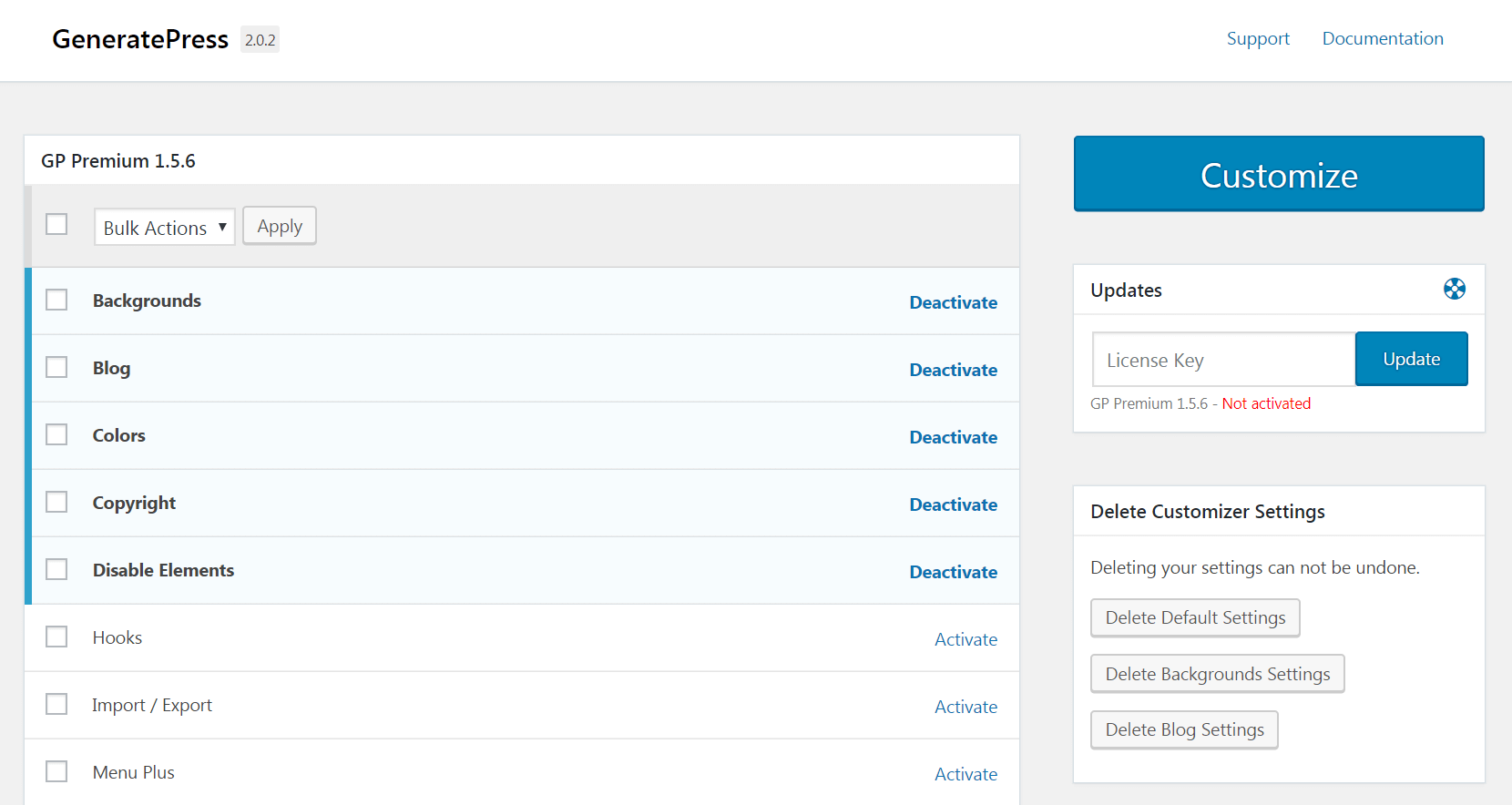The image depicts a settings page for the GP Premium 1.5.6 plugin, likely on a WordPress site. The interface is filled with technical jargon and various options, which may be initially confusing. Prominent among the options are terms like "background," "blogs," "colors," "copyright," "disable elements," "hooks," "import," and "menu plus." On the right side, there is a large blue button labeled "Customize," intended for further tweaking the site's appearance. Below that, there is a section for inserting a license key, implying that the current installation may be on a free trial or not fully activated yet. Additional options include the ability to delete customizer settings, with explicit warnings that such actions cannot be undone, affecting settings related to backgrounds, blogs, and possibly other site elements. Overall, the image highlights the extensive customization capabilities of the plugin, aimed at allowing users to modify various aspects of their WordPress site's design and functionality.